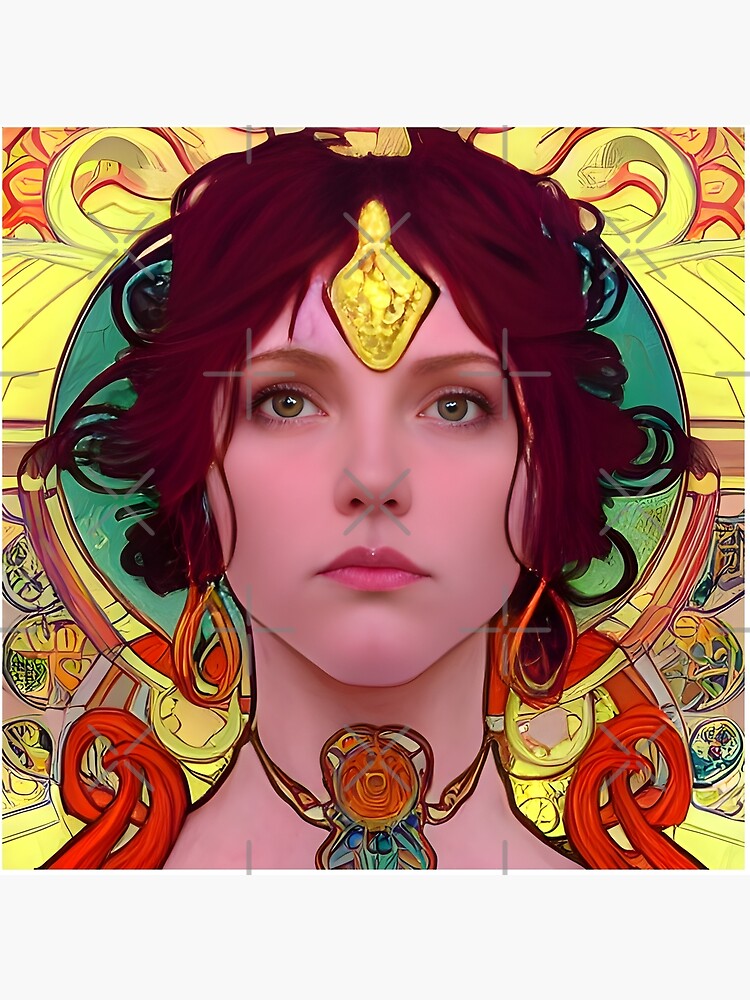This mixed-media photograph portrays a young woman with a striking face gazing straight ahead. Her face is rendered photographically with slightly colorized, pink-toned skin, adorned with pink lipstick, brown eyebrows, and subtle makeup. She sports vivid red, curly hair that appears painted on. Accentuating her face are round gold earrings and a rosebud choker, complemented by a large, prominent gold jewel on her forehead. The background is an intricate, stained glass-like pattern in a vibrant palette of yellow, blue, green, and gold. Encircling her head is a teal to green gradient circle that brings focus to her serene expression. Overlaying the entire image are transparent watermarks consisting of X's and crosses, adding a unique texture to the composition.